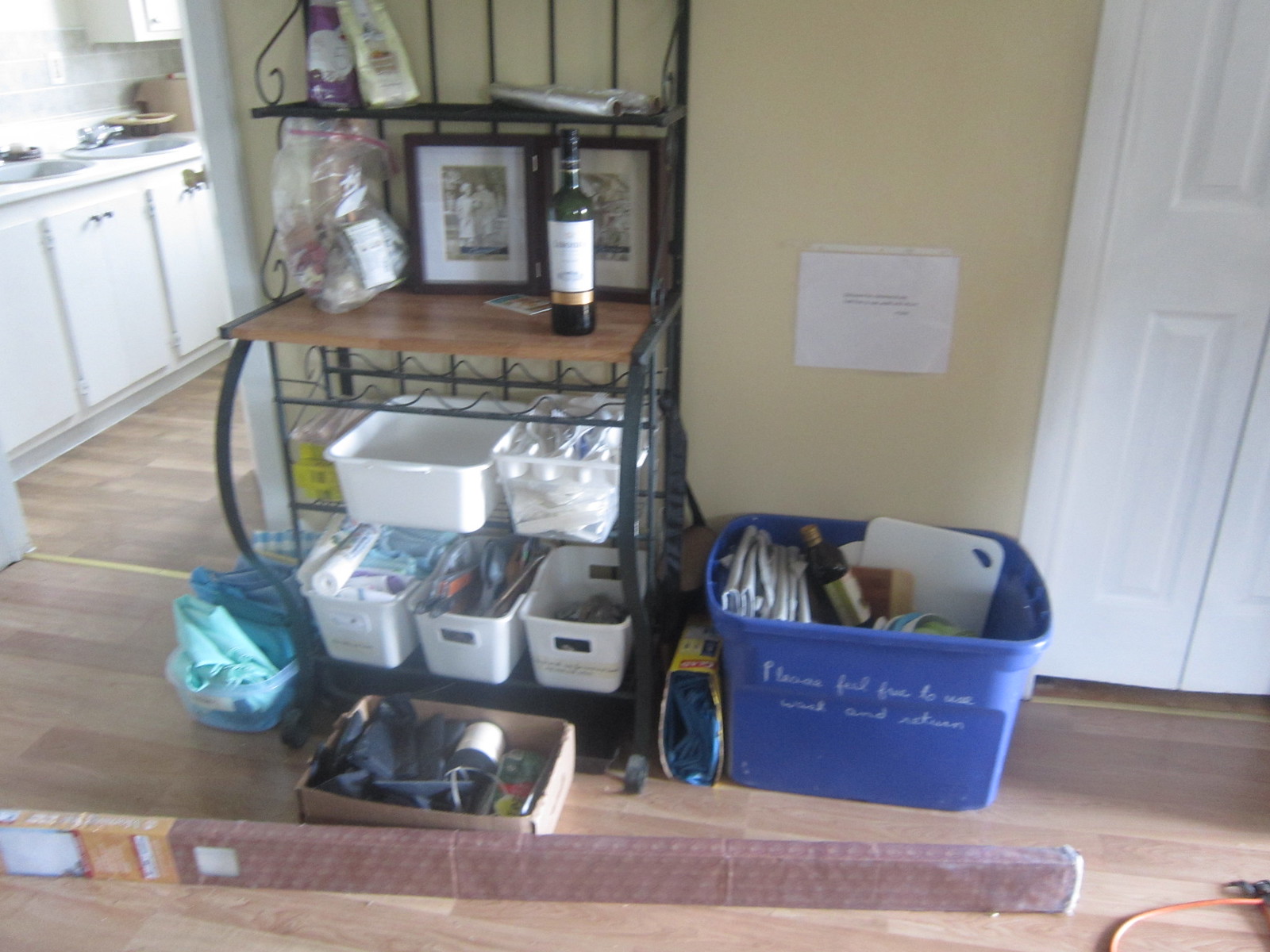The image depicts a storage area adjacent to a kitchen, characterized by an eclectic assembly of items and containers. Central to the scene is a metal rack, featuring a bottle of wine prominently displayed on a wooden shelf. Above the wine bottle, more items can be seen, accompanied by old photographs placed on the same level. The wooden shelf is pressed against a tan colored wall, contrasting with the surrounding white doors and moldings.

To the side of the metal rack sits a blue tub filled with various miscellaneous items, which include a bottle and a cutting board. Directly below the shelf holding the wine bottle and pictures, five bins are stacked, each containing an assortment of miscellaneous objects. In front of the rack lies a short cardboard box, also stuffed with various items.

To the left of this setup, a container holding several light blue bags can be observed. Additionally, prominently situated in front of everything is a long maroon-colored box, adorned with pictures at one end, extending approximately five feet in length. All items rest upon a light-colored wooden floor, adding to the overall warm and rustic feel of the storage area.